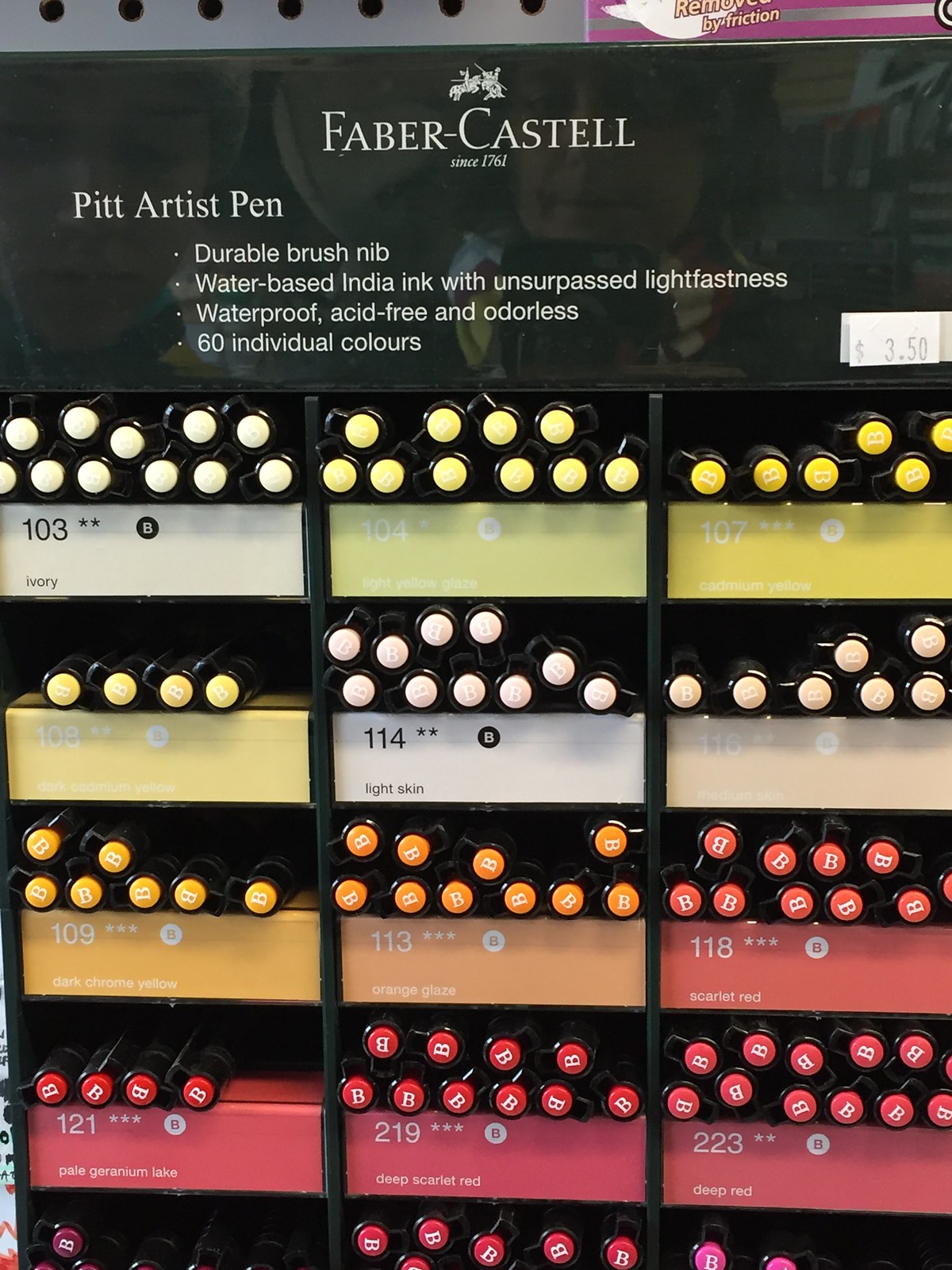This image captures a detailed and well-organized display case in what appears to be an arts or crafts store. At the top of the black background display, the text reads, "Faber-Castell since 1761" followed by "Pitt Artist Pen durable brush nib water-based India ink with unsurpassed lightfastness, waterproof, acid-free, and odorless." Below this text, the display boasts 60 individual colors, each neatly arranged in five rows with three columns of little cubbies. 

Every cubby holds pens with the corresponding color visible at the tip, and each pen is individually numbered with its specific hue marked beneath. The first pen is marked 103 and labeled as ivory, followed by a range of colors including light green, yellow, a darker yellow, and various shades of beige, white, orangey-red, peach-orange, yellowy-orange, and different shades of red. The exacting organization and clear labels make it easy to see and choose the desired color, showcasing the vibrant and diverse palette offered by Faber-Castell.